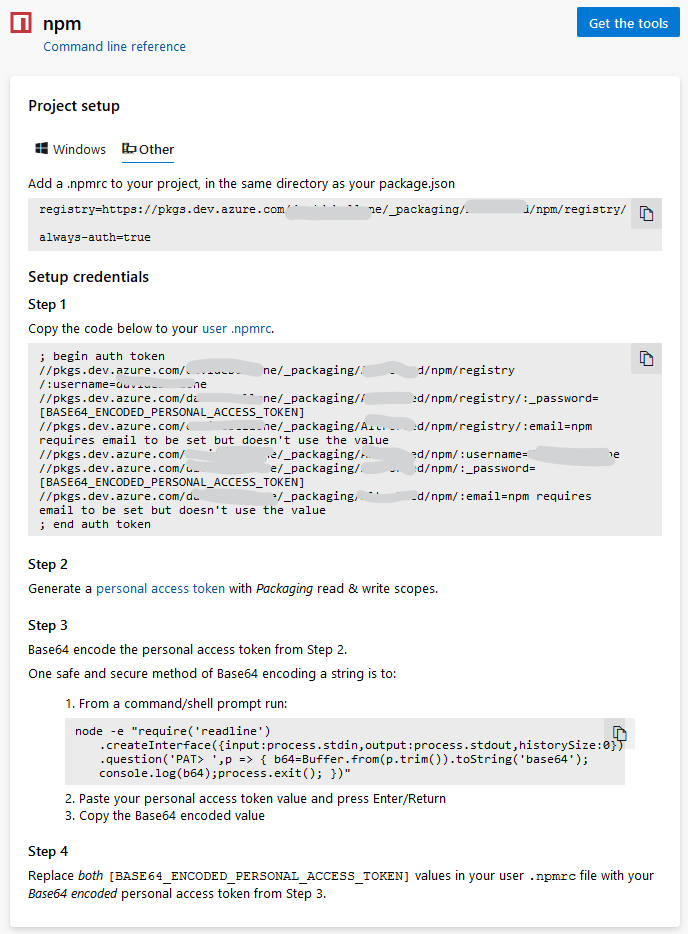**Caption:**

A screenshot captures a structured layout of a website's code information interface. The image has a white main body framed by a light grey border. Within the main body, there are three light grey blocks containing various code segments and instructions. 

In the top left corner, a red block features a stylized 'N' for November, adjacent to bold, lowercase text that reads "N for November, P for Papa, M4 Mike." Below this, "command line reference" is highlighted in blue. The top right corner includes a blue button labeled "Get the Tools" in white text.

The central part of the image has a white block with the headline "Project Setup" in the top left. Beneath the headline, there are options for "Windows" and "Other," with "Other" currently selected. This section includes detailed technical instructions.

The first instruction is to add an `.npmrc` file to your project directory along with your `package.json`. Following this, a grey block showcases a segment of code.

Below the grey block, in the white section, it states "Setup Credentials". The first step instructs users to copy a provided code into their user `.npmrc`. Another grey block follows, displaying the code to be copied.

Step two advises generating a personal access token with packaging read and write scopes. Step three involves base64 encoding the personal access token obtained in the previous step. A subsequent grey block contains further steps.

Step four instructs users to replace specific technical token values in their user `.npmrc` file with the encoded personal access token generated in step one.